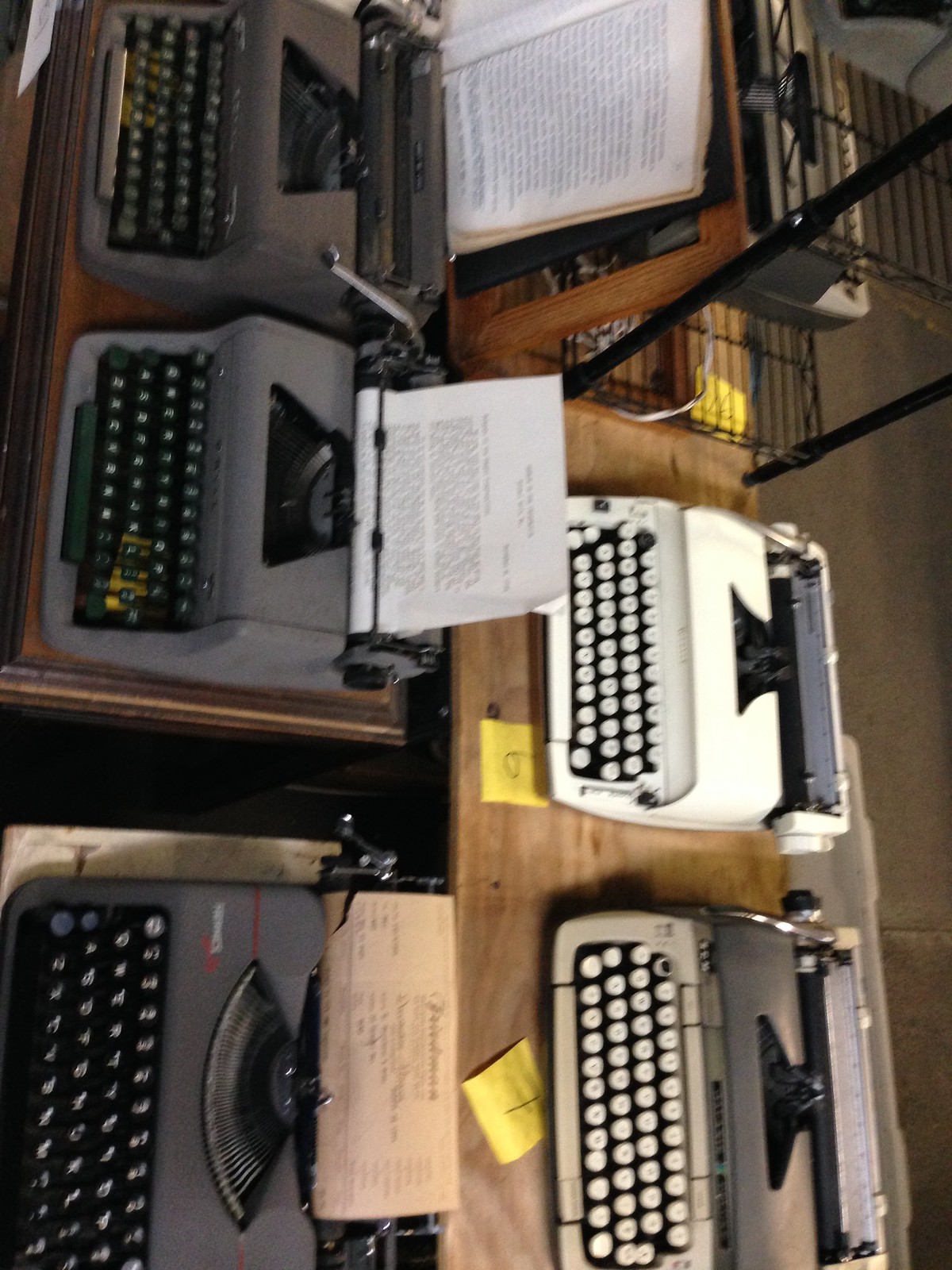This sideways color photograph, taken from a roughly 15-degree overhead angle, captures a collection of five vintage mechanical typewriters arranged in two rows, all oriented in the same direction. On the far right sits a white typewriter adorned with a yellow post-it note labeled "6." To its left, a light brown typewriter has a yellow post-it note marked "7." Moving leftward, there is a black typewriter containing a yellowed sheet of paper. Above this, a gray typewriter holds a white sheet of paper with text. At the very top, another typewriter in charcoal gray completes the lineup. Additionally, an open book is positioned above one of the typewriters, suggesting that users could transpose its content onto the typing sheets. The typewriters, reminiscent of 1960s business models, seem to be part of a sale or auction, as indicated by the numbered post-it notes.